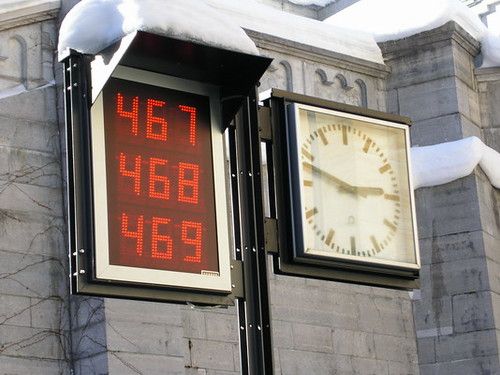This outdoor photograph captures a unique concrete brick structure, reminiscent of a castle with its gray, imposing facade. The top of the building is obscured from view, adding to its enigmatic charm. The entire edifice is blanketed in white, leaving viewers to ponder whether it is an artistic paint job or a layer of freshly fallen snow. Despite the snowy appearance, the day is bright and sunny, casting a pleasant ambiance over the scene. Prominently displayed on one wall of the building is a square clock, distinguished by its lack of numbers and simple black hands. Adjacent to this analog clock is a digital display featuring the red numerals 467, followed by 468, and then 469, arranged vertically in a column. The juxtaposition of the timeless analog clock and the modern digital readout adds an intriguing contrast to the otherwise monolithic structure.